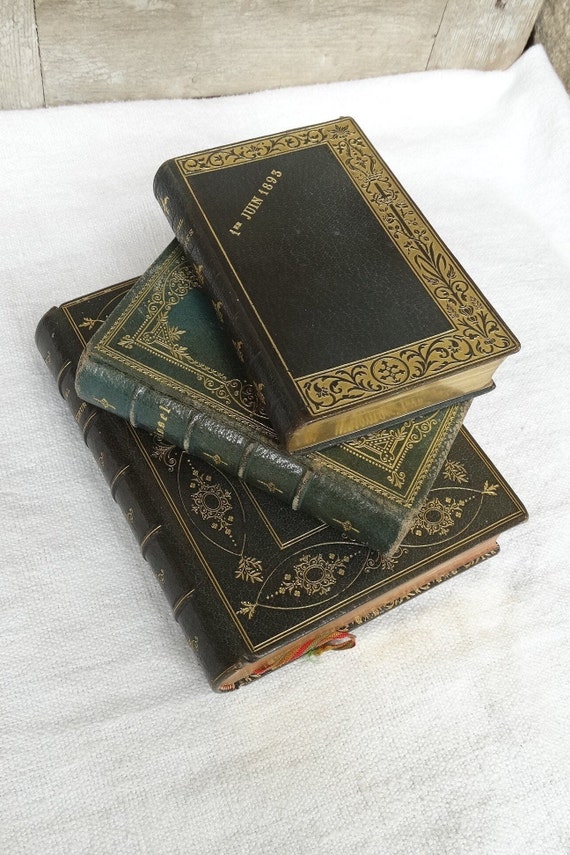The photograph captures a detailed close-up of a stack of three antique books arranged on a white fabric backdrop. The composition features one black book at the bottom, which is the largest, showcasing intricate gold patterns on its cover and spine. Above it lies a green book, slightly angled to the left, adorned with delicate gold floral designs on its cover and spine. The smallest book rests on top, also black with a gold decorative border along three edges, and a clear gold inscription on the cover that reads "J.U.I.N. 1893". The clarity of the image is exceptional, with bright, even lighting highlighting the fine details of the books' worn and vintage appearance. The stack is centered against a subtle background, creating a vivid portrayal of these old, ornate volumes.